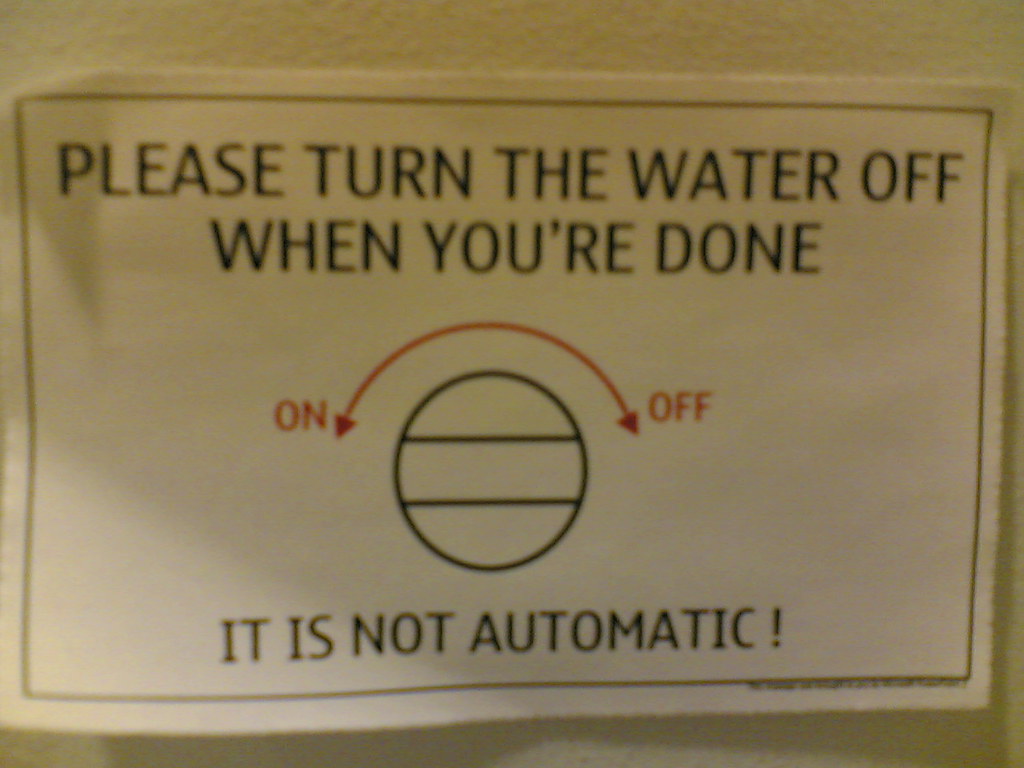This photograph captures a computer-printed warning sign affixed to a textured white wall. The sign, framed by a black border, consists predominantly of black text with some red elements. The main text urges readers to "please turn the water off when you are done," emphasizing that "this is not automatic" with a notable exclamation point at the end. A red, two-sided curving arrow illustrates the directions, indicating "on" to the left and "off" to the right, accompanied by a black circle with two horizontal lines representing a dial or knob. The sign appears to be printed on inexpensive printer paper, and there's a blurry signature or logo in the bottom right corner, possibly alluding to the owner or a website. The setting suggests a place like a laundromat where manual water control is necessary.